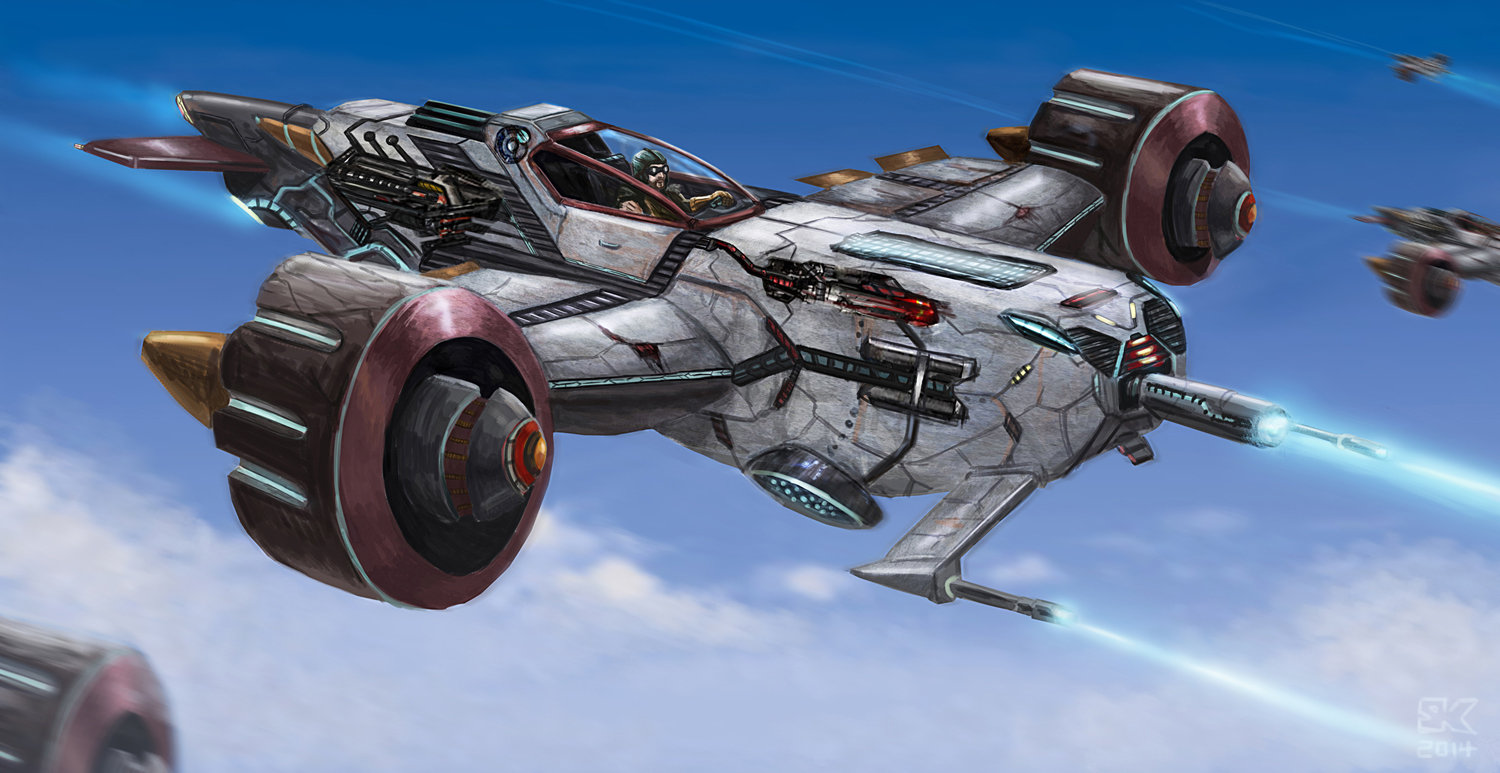This image portrays a dynamic science fiction aerial dogfight set against a picturesque, Earth-like backdrop with a blue sky and scattered white clouds. Dominating the scene are several futuristic aircraft, reminiscent of designs from Star Wars but adapted to atmospheric flight. The central aircraft features imposing turbine engines mounted on the tips of its wings, which flank a purple cockpit where a bearded pilot in a helmet and goggles sits. The aircraft appears to be heavily armed, with a prominent laser cannon at the front and two additional laser guns beneath the nose, all emitting vivid blue beams.

Distinctive patterns of fine line breakage, as if the hull has cracked like an eggshell, crisscross the aircraft's surface, revealing underlying metal piping and inner cables where panels have fallen away. This detail is complemented by streams of smoke trailing from the engines, emphasizing the craft's high-speed maneuvering.

Additional futuristic fighters blur in the background, suggesting rapid motion and intensity in the airspace. One of these is partially visible with just its turbine engine peeking from the lower left corner while two more flank the central fighter, all moving towards the right side of the image. The vivid scene, rich in details and action, is rendered as a detailed drawing, bringing the thrilling atmosphere of a high-stakes dogfight to life.